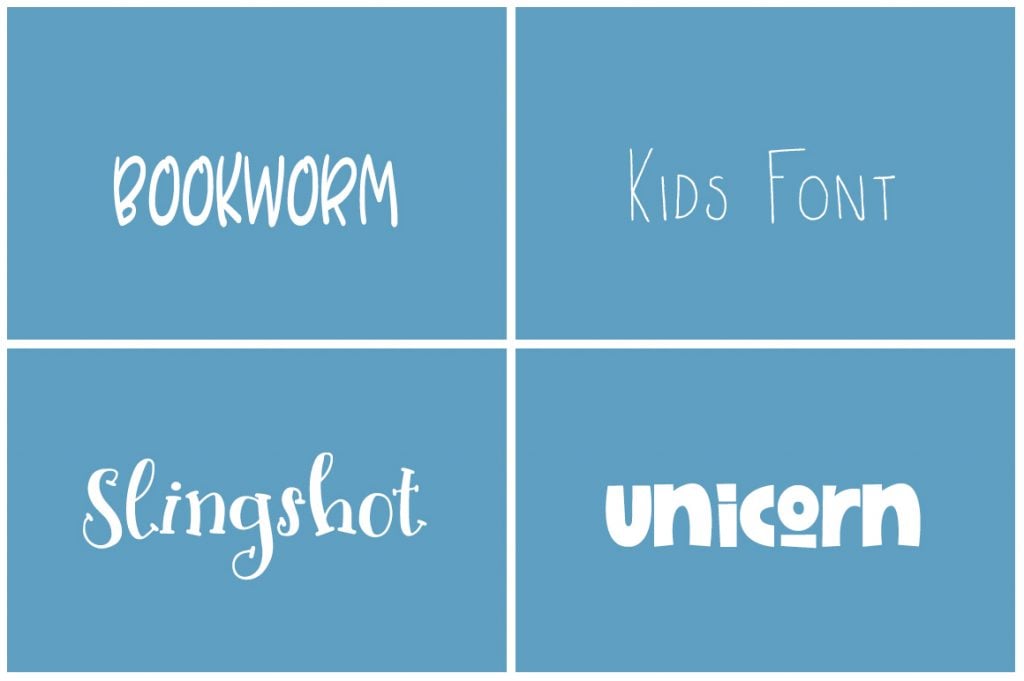The image features four medium-blue rectangles arranged in a grid layout, with two on the top row and two on the bottom row, separated by a prominent white line. Each rectangle showcases a different font face, exemplifying diverse typography styles. 

In the top-left rectangle, the "Bookworm" font is displayed in all capital letters. This font has a bulky, hand-drawn appearance, giving it a bold and distinctive look. 

The top-right rectangle features the "Kids Font," characterized by very thin, angular, hand-drawn lines. This font is also presented in all caps, offering a simple and straightforward aesthetic.

On the bottom-left, the "Slingshot" font adds a touch of elegance with its frilly and fancy design. This font includes little serif bits at the ends of the letters, making it reminiscent of chalkboard writing often seen in cafes.

Finally, the bottom-right rectangle displays the "Unicorn" font in lowercase letters. This font is chunky and bulky, standing out with its robust and playful appearance. 

Each font name is clearly attached to its corresponding style, providing a comprehensive visual reference for different typographic expressions.